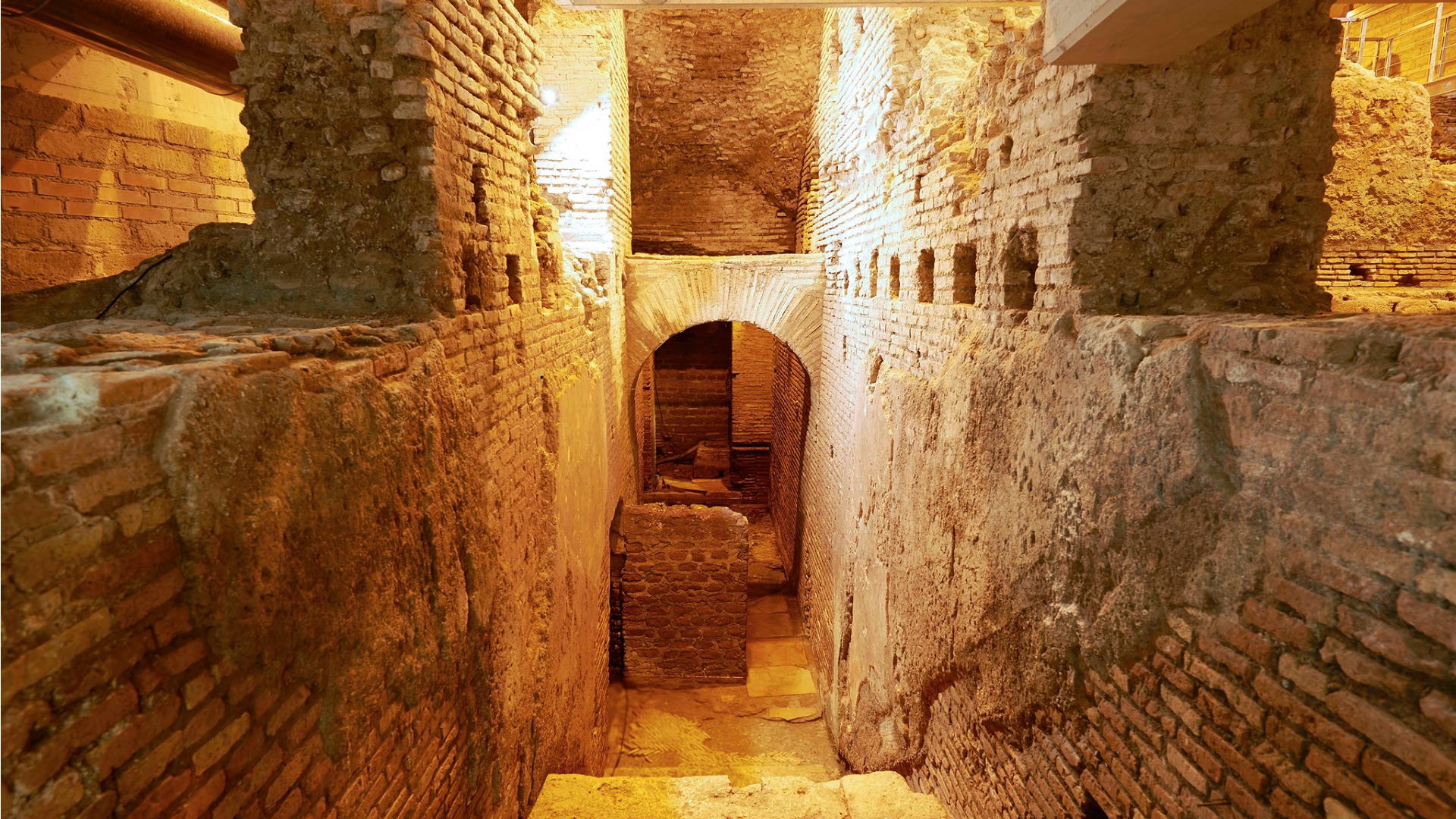The image depicts a scene set within an ancient, dungeon-like area reminiscent of an old castle or catacomb. The foreground features a staircase made out of sandy, yellow-toned stones or cement, leading downwards into a deeper section of the structure. These stairs are bordered by walls constructed from bricks that appear yellowish due to ambient lighting, though hints of red and tan bricks are visible towards the front. The walls are partly covered in a crusty, aged material, adding to the historical ambience. 

Above and around the staircase, intricate architectural details are visible, including an ornate doorway with a rounded arch. On the right side, white pipes run along the top corner of the wall, while the left side receives light casting a warm yellow hue. Further down the corridor, the tunnel extends into what appears to be a wooden or plank-covered floor. A four-foot-high brick structure stands along the path. At the end of the tunnel, there is a brownish door, framed by the same yellowish bricks seen throughout. The entire setting evokes the feel of an ancient, possibly Egyptian-influenced structure with its unique and historically rich design elements.